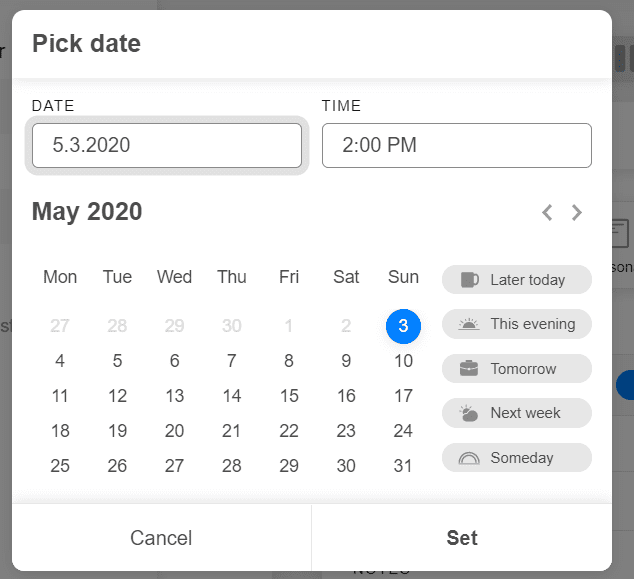This detailed image captures a screenshot of a pop-up window featuring a calendar interface. The calendar itself is displayed against a white background and is labeled "Pick Date" at the top left. Below this title, there are two sections: the left section specifies the date as "5.3.2020", and the right section specifies the time as "2 PM". The calendar view underneath these sections is set to May 2020.

Adjacent to the calendar on its right, there are five grey, pill-shaped sections, each containing an icon on the left side of the pill and corresponding text on the right side, positioned inside the grey bubble. The entire layout is focused on presenting a user-friendly interface for selecting specific dates and times.